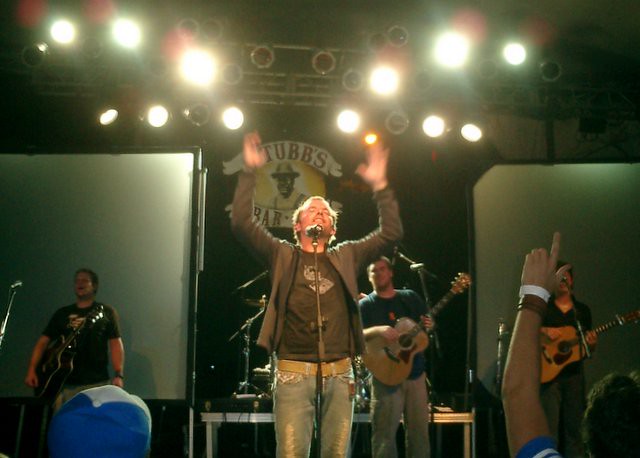In this rectangular photograph, we see a dynamic concert scene taking place at Stubbs Bar. The image captures a Caucasian lead singer, prominently positioned in the center of the stage, from the knees up. He is passionately performing with his arms raised, eyes closed, and looking upwards. He sports pale blue jeans, a tan belt, and a black t-shirt with a white design, layered with a black, long-sleeve leather jacket. 

To his left, a guitarist in a green shirt holds a light brown acoustic guitar. Slightly obscured behind him and to the right stands another guitarist in a blue t-shirt paired with light blue jeans, also gripping an acoustic guitar. In the background, a drum kit is partially visible, set up on a metallic frame but largely hidden by the performers in the foreground.

The stage is illuminated by intricate lighting: two arcs of mostly white spotlights frame the stage from the top left and right, converging toward the bottom center. Six horizontal lights, divided into two sets of three, stretch across the middle.

In the audience, a hand rises in the foreground on the right side, pointing upward with thumb and index finger extended. The hand belongs to a person in a red and blue striped shirt, accessorized with white and black bracelets. The whole scene is set against a predominantly dark backdrop, enhancing the brilliance of the stage lights and the vibrant energy of the concert.